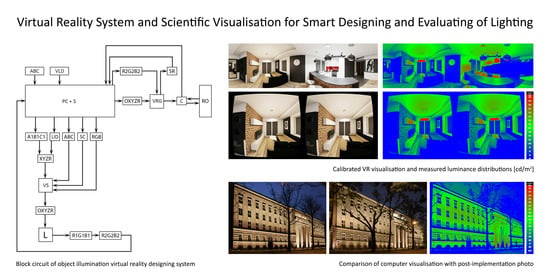An elaborate diagram titled "Virtual Reality System and Scientific Visualization for Smart Designing and Evaluating of Lighting" spans the left third of the image. This section presents a complex block circuit diagram for object illumination within a virtual reality design system, featuring numerous interconnected rectangles and arrows, with text too small to discern. The right two-thirds of the image contains a series of photographs that illustrate lighting evaluations in various environments. At the top, four side-by-side images depict an office interior: two show the office in normal color and two in a night vision-like, heat map style with blue, green, and occasional red hues, highlighting luminance distributions. Below these, three additional images focus on the exterior of a large brick building—likely a university—during nighttime: one in regular color, one altered, and the last in a similar blue-green heat map format. The text under these visuals denotes "Calibrated VR Simulation and Measured Human Distributions," emphasizing the system's capability to analyze and visualize lighting effects comprehensively.